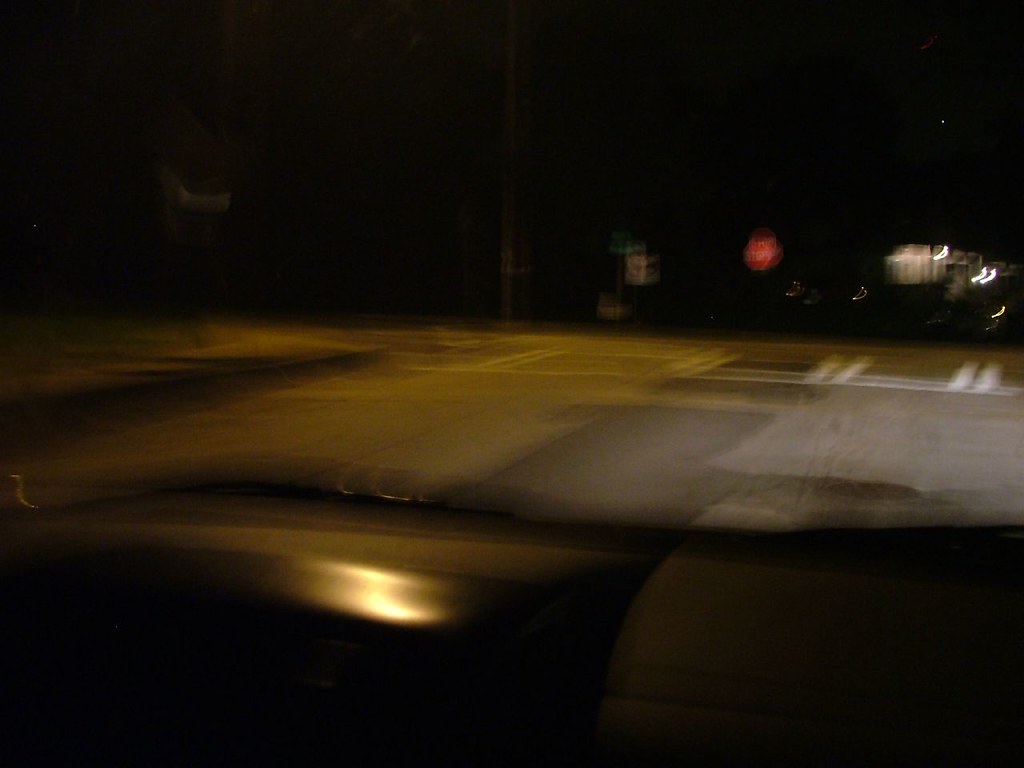A dimly lit parking lot at night is captured from the interior of a car. The view through the windshield, with its visible window wiper, reveals a dark expanse primarily shaded in gray and black. In the distance, a series of white squares, likely parking space markers, can be seen faintly illuminated. A prominent red round sign stands out, accompanied by a green square sign on a pole nearby. To the right, a white sign is visible, under the soft glow of several white lights. A bright white light hangs in the night sky, adding a celestial touch to the scene. The car's shiny black and gray dashboard is partially visible in the foreground, and its headlights cast a stronger illumination on the right side of the parking lot, creating a stark contrast with the darker left side.